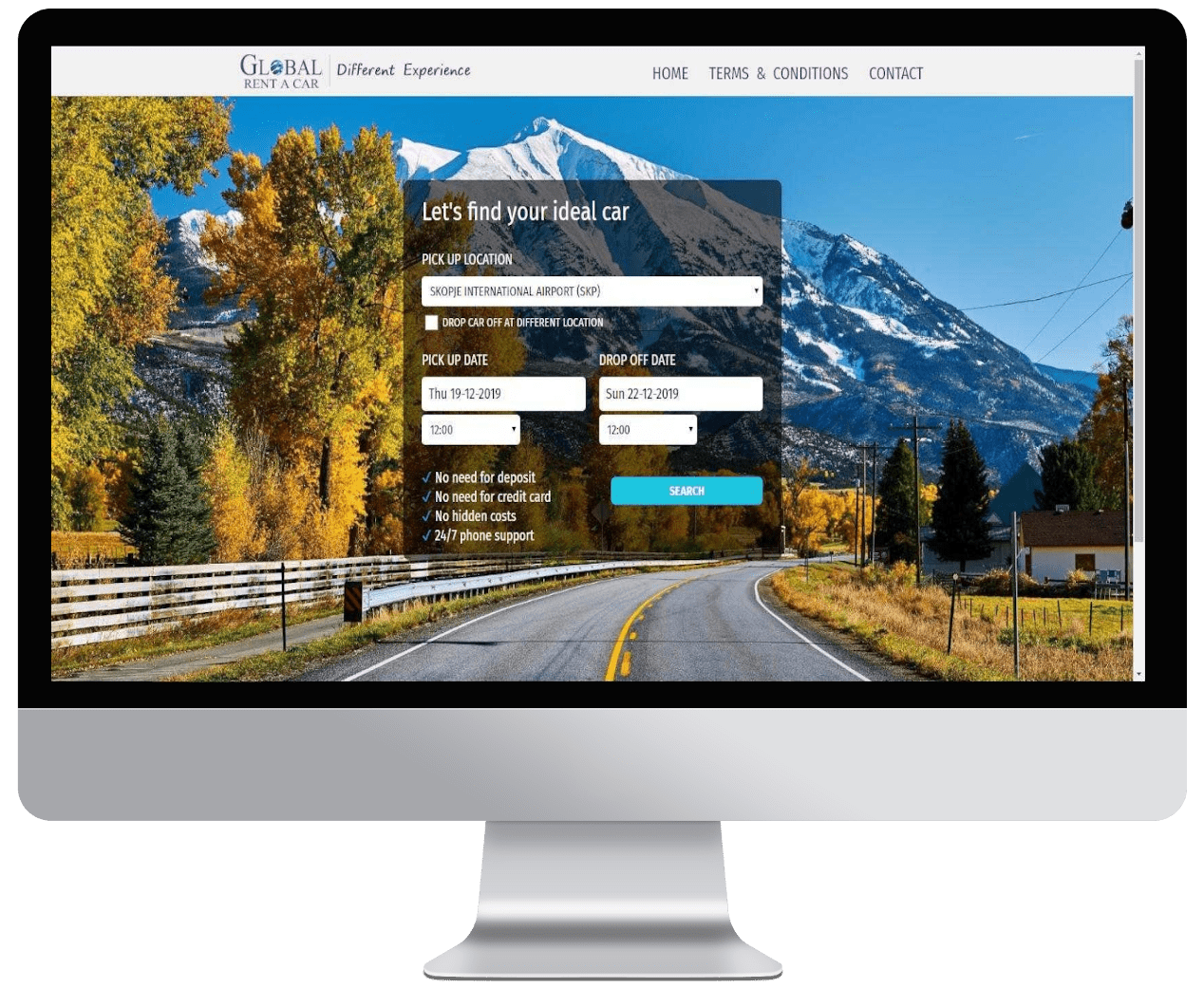In this image, we see a digital interface which appears on either a keyboard or a computer screen, possibly a large MacBook or an iPhone. The user interface has a streamlined design beginning with a top navigation bar labeled "Global." 

At the bottom right corner, there is a button labeled "Different Experience" alongside navigational icons. The interface includes sections titled "Trends and Conditions" and "Contacts." The background of the main header features a scenic road flanked by trees in autumn foliage, leading towards snow-capped mountains in the distance.

Central to the display is a prominent call-to-action button that says, "Let's find our ideal car." Directly beneath this, the words "Pickup Location" appear above a text input box with a white background reading "International Airport." Adjacent to this is a checkbox with the option "Drop Car at Different Location."

Further down, there are two dropdown menus labeled "Pickup Date" and "Drop Off Date," which are pre-set to dates such as Sunday, the 22nd. The interface concludes with a distinctive blue switch bar at the bottom.